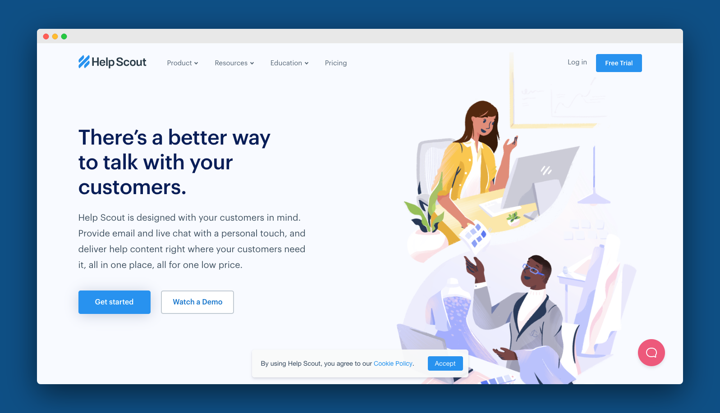A webpage for Help Scout is displayed prominently. To the right-hand side, approximately two-thirds of the way across, there are vibrant graphics depicting two individuals engaged in communication. In the first graphic, a woman with medium skin tone, shoulder-length brown hair, and wearing a cheerful yellow sweater, is seated at a desk intently looking at her monitor. Her left hand is raised as if she is gesturing or conversing, suggesting an active interaction, possibly with someone on the screen or with the illustrated figure below her.

The second graphic features a dark-skinned man adorned with stylish blue glasses, dressed in a sophisticated suit accented by dark blue lapels. The scene portrays him as a potential recipient or partner in this dialogue. 

Above these engaging visuals, the text header reads, "Log In | Log Out." Directly below, a message stands out in bold lettering: "There’s a better way to talk with your customers." The accompanying description highlights Help Scout's customer-centric design, emphasizing the platform's ability to provide email and live chat services with a personalized touch. It assures users that Help Scout delivers help content precisely where and when customers need it, consolidating these services in one seamless experience, all offered at an affordable price.

At the bottom, two call-to-action buttons invite users to "Get Started" or "Watch a Demo," encouraging them to explore Help Scout's features and benefits further.